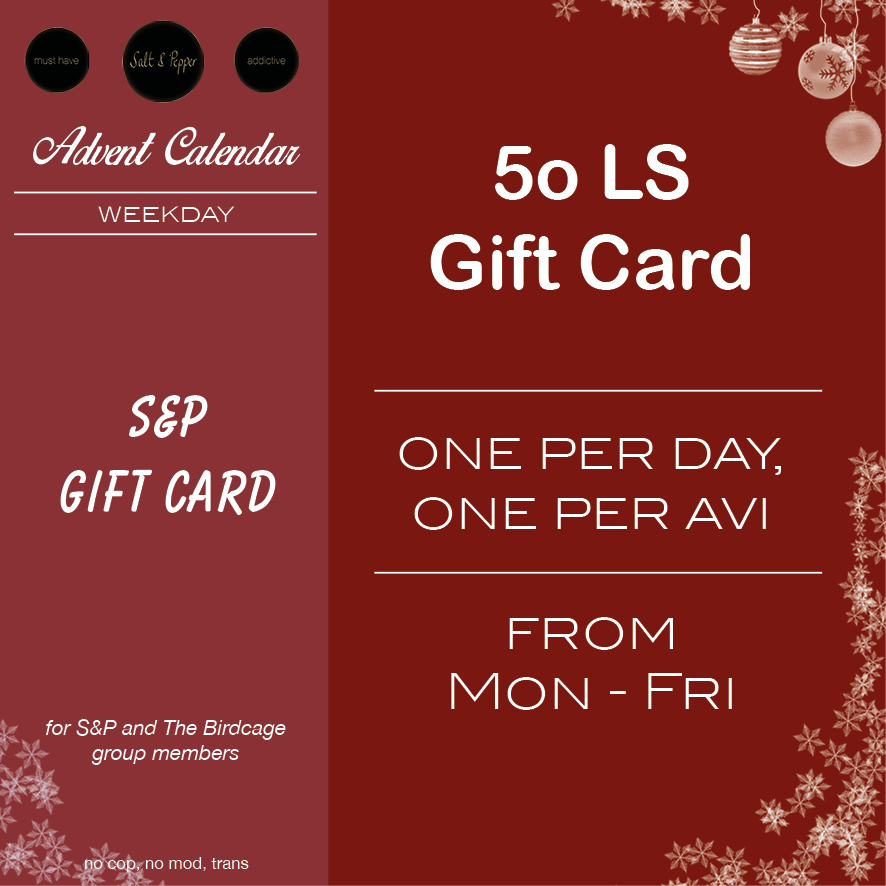The image depicts a festive advertisement, primarily in red, with "Advent Calendar Weekday" written in white font at the top left corner. Above this, the title "Salt and Pepper" is encased in a black circle. The central theme promotes a "50 LS Gift Card," with the policy of one card per day, one per avatar (AVI), available from Monday to Friday. It specifies that the promotion is for S&P and the Birdcage group members. Key phrases such as "No comp, no mod, trans" are noticeable, alongside decorative elements including snowflakes at the bottom right corner and ornaments with additional snowflakes at the upper right. The bottom left features text confirming this offer is exclusive to S&P and the Birdcage groups, and the black circles contain motivational or descriptive phrases like "must have," "addictive," and "Salt and Pepper."